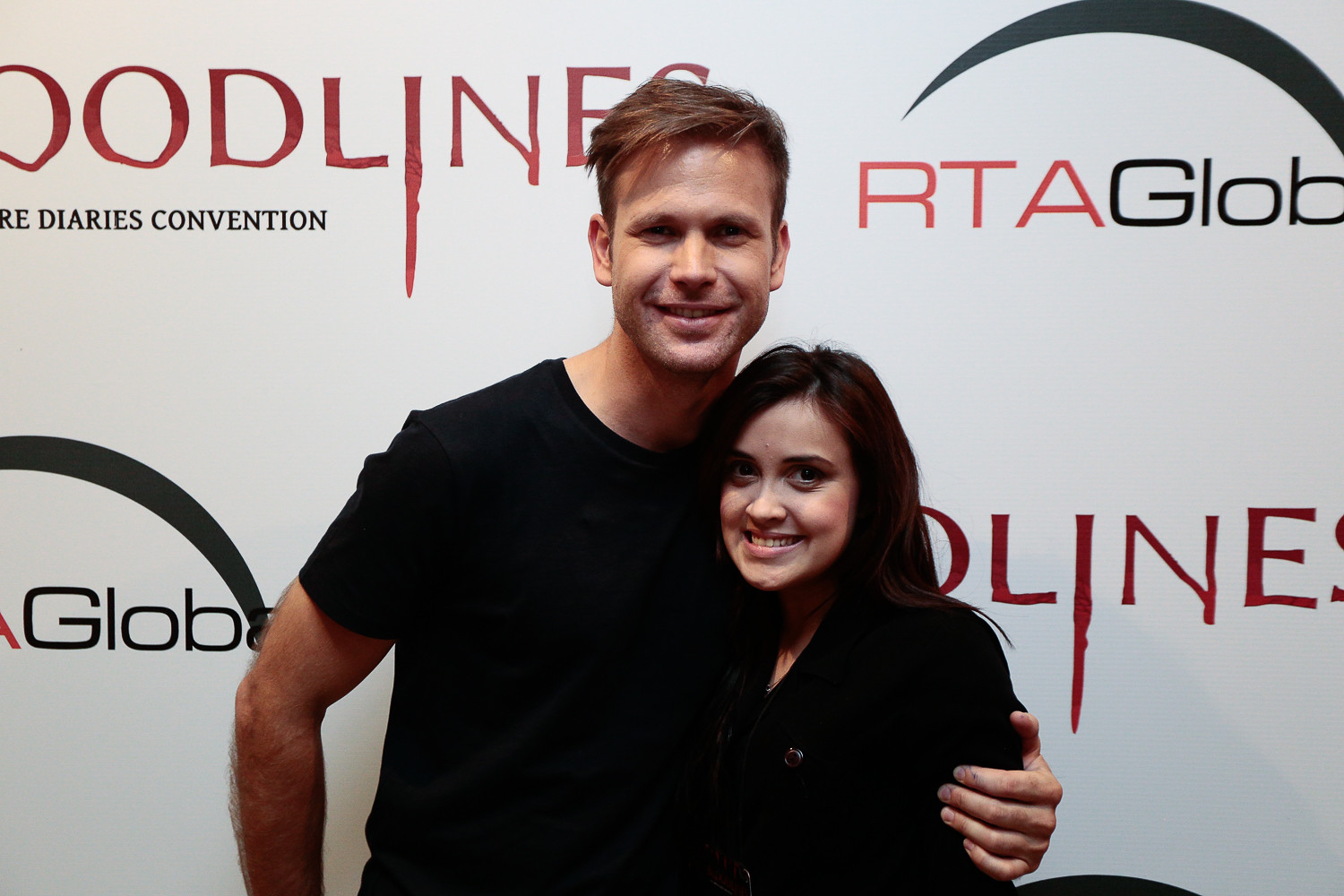This image features a man and a woman standing together in front of a step-and-repeat backdrop, presumably at a red carpet event or premiere. The backdrop has a white background adorned with various logos and texts. One prominent logo reads "BLOODLINES" in bold red letters, and another part of the text includes "RTA GLOBAL." Although some of it is obscured, the words "DIARIES" and "CONVENTION" are also visible. The man has reddish-brown hair parted to the side and is wearing a black crewneck t-shirt. His left arm is around the woman, who is smiling and dressed in a black jacket. She has long, dark, brownish hair. The man is identified as an actor from "The Vampire Diaries" series, portraying the character Alaric, while the woman appears to be a fan taking a photo with him.